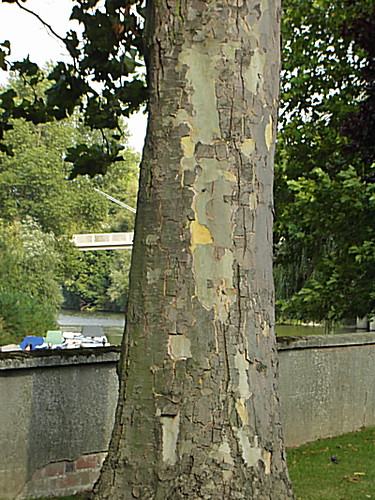The photograph, taken on a cloudy day, captures a close-up of an old tree trunk, likely a sycamore or oak, situated in a lush green grassy area. The focal tree shows significant wear, with much of its bark peeling off to reveal a yellowish inner layer. Hanging from the tree, typical sycamore or oak leaves are visible, indicating its healthy green foliage. In the background, an array of green trees forms a verdant backdrop. On the left, moored boats can be seen on the water partially obscured by a low concrete wall, which shows wear at the base revealing underlying bricks. A white bridge spans across the dark greenish water further back, completing the picturesque outdoor scene.